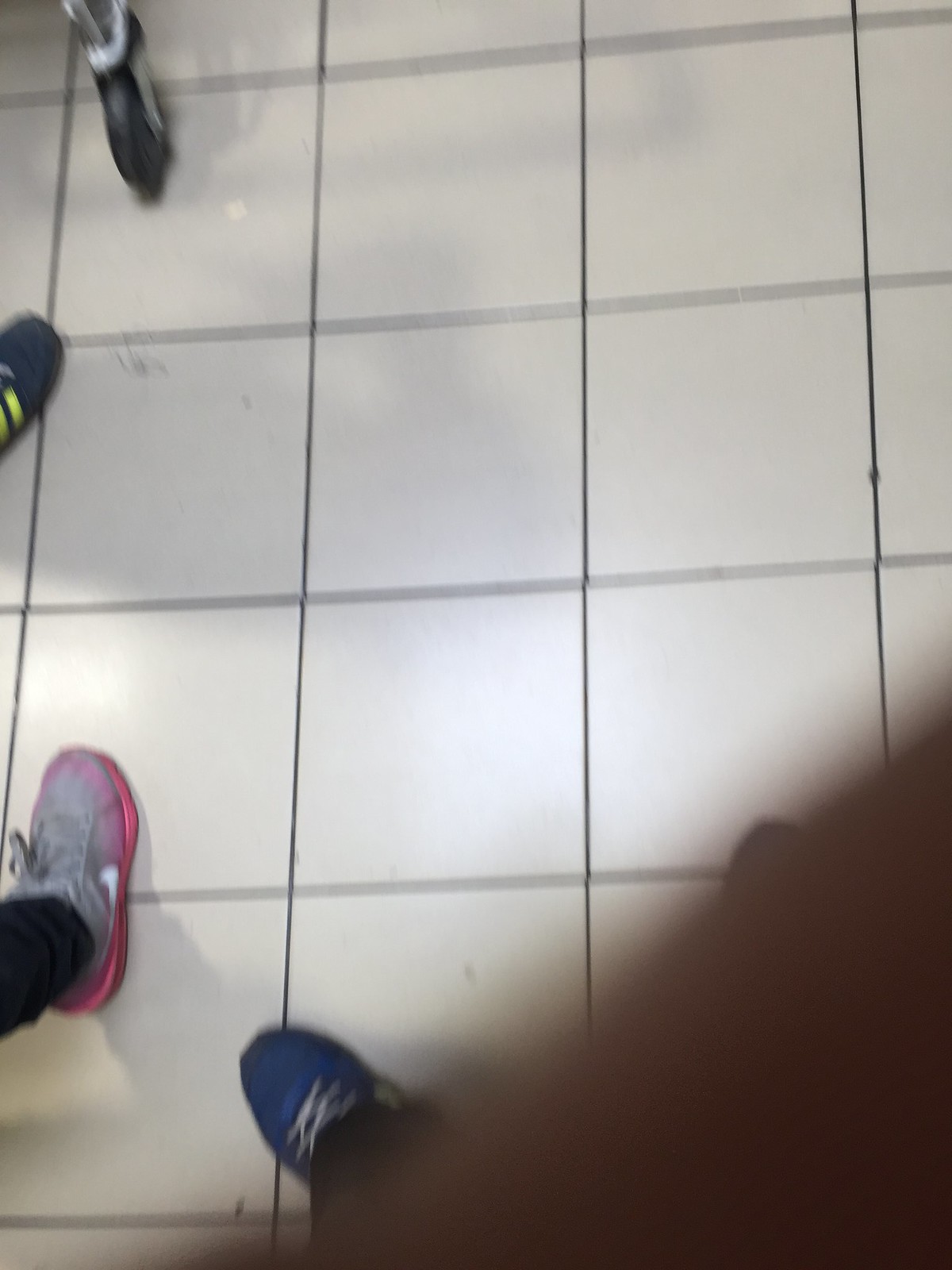This image captures a top-down view of a grocery store floor. The flooring consists of beige or white tiles, separated by thin black grout lines. A black wheel attached to a silver mechanism appears in the top left corner, with a vertical bar extending from it, likely part of a shopping cart. In the bottom right, part of a person's arm is visible, albeit blurred, alongside two partially shown shoes. The shoe on the left is blue with white shoelaces, and to its left is another person's ankle clad in gray pants, wearing white Nike shoes with a pink base, featuring the iconic white Nike swoosh. In the top left corner, another shoe can be seen, dark blue with yellow stripes, reminiscent of 1980s footwear.